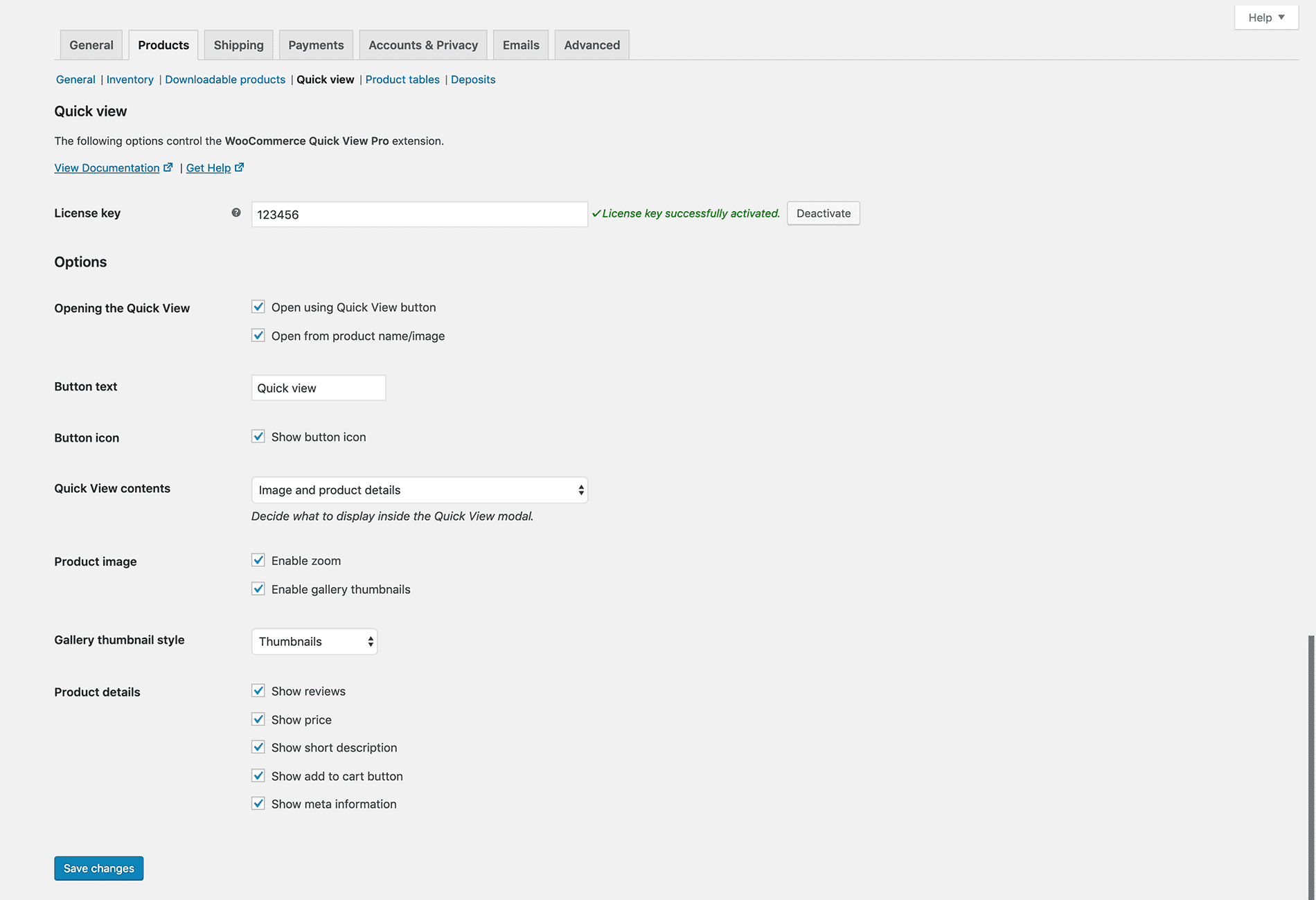In this detailed screenshot set against a light gray background, we observe an intricate interface with exceptionally small text. At the top, a menu bar presents several tabs arranged from left to right, labeled: General, Products, Shipping, Payments, Accounts and Privacy, Emails, and Advanced. Positioned in the top right corner is a Help button.

The prominently opened Products tab reveals a sub-menu area that includes additional options: General, Inventory, Downloadable Products, Quick View (highlighted in black), Product Tables, and Deposits, all listed from left to right.

Directly beneath the highlighted Quick View tab, there's a section titled 'License Key' which contains a field designated for entering a key. Further options below this field within the Quick View include two choices: "Open using Quick View button" and "Open from Product Name and Image," both of which are marked with checkmarks.

Towards the bottom, more detailed elements are listed, such as 'Button Text Boxed,' 'Button Icon,' 'Quick View Contents,' 'Product Image,' 'Gallery Thumbnail Style,' and 'Product Details.'

A functional blue button labeled "Save Changes" is positioned in the lower left corner, signifying an option to save any modifications made within this section.